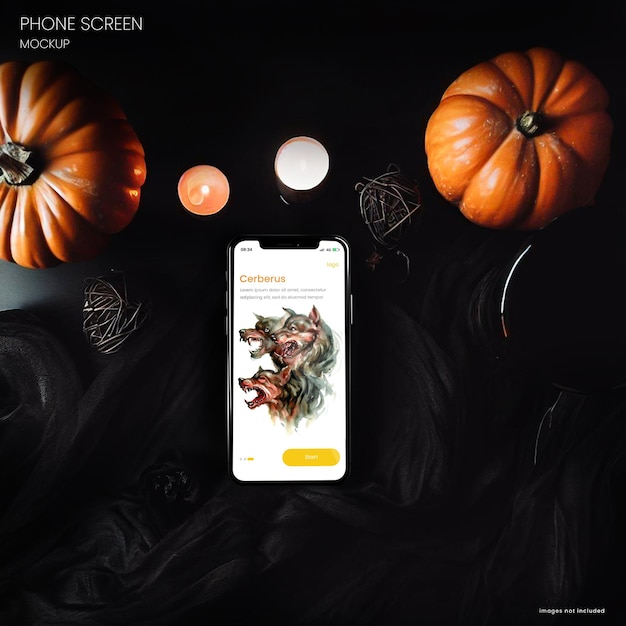The image depicts a top-down view of a dark-themed setting featuring an autumnal or Halloween arrangement. At the center, there is a mock-up of a smartphone screen with a white background. The screen displays the word "Cerberus" in yellow text at the top. Below this, there are two lines of placeholder Latin text followed by an image of three snarling wolf heads painted together. At the bottom of the screen, there is a button labeled "Start."

Flanking the smartphone are two pumpkins—one on the left and one on the right. The left pumpkin is partially illuminated by a soft light, while the rest of the scene remains in shadow. Above the smartphone, there are two lit candles: the left candle is orange and the right candle is white. Alongside the candles are two small balls made of metal twine, adding a touch of rustic charm to the composition.

The overall atmosphere is moody and evocative, suggesting a mystical or eerie theme. The subtle lighting highlights the pumpkins and candles, drawing attention to the central phone screen mock-up and its enchanting content.